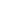The image depicts a dark gray Audi four-door vehicle driving on a snow-lined highway through a dense forest of lodgepole pine trees. The snowy landscape extends up to the edge of the roadway, which has been plowed. The Audi is in motion, creating a slight blur in the background, enhancing the sense of speed and movement. The car features dark gray wheels, a black front grille, and its lights are on despite the daylight. A license plate reads CD228RX, and the car bears the logo and words "Add Driving Academy" on its side, indicating it’s likely being used for driving instruction. No other vehicles or people are visible in the clear, naturally lit setting. The overall high-quality image gives a commercial-like feel, emphasizing both the vehicle and the serene, wintry environment.